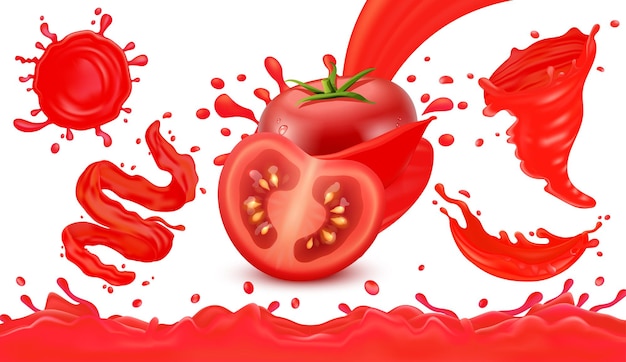This digital illustration features a vivid and striking display of tomatoes and tomato-related imagery, set against a stark white background. At the center is a whole tomato with a green stem, positioned behind a halved tomato that reveals its seed-filled interior. Surrounding the central tomatoes are various fluid elements resembling tomato juice or sauce. Along the bottom of the image flows a river of tomato juice, while in the top left corner, there is a circular splotch of tomato juice. To the left, there is a ribbon-shaped flow of the red liquid. On the right side, there's a dynamic swirling shape akin to a tomato juice tornado, along with an additional splotch resembling the bottom part of someone's lip. The image's composition, with its numerous red splotches and flowing elements, gives the impression of an energetic burst, possibly linked to an advertisement for ketchup, tomato sauce, or a similar tomato-based product.